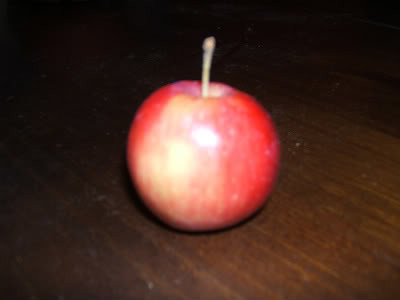A small, bright red apple sits on a dark brown wooden surface that has subtle green undertones running diagonally. The photograph captures the apple at a slight angle rather than straight on, giving it a dynamic perspective. On the front of the apple, there's a noticeable reflection caused by the camera's flash, creating a light spot on its glossy skin. The top of the apple dips inward, revealing a surprising touch of purple in the far part of the dip. A straight, green stem protrudes vertically from this dip. The background of the image is pitch black, providing a stark contrast that accentuates the vibrant colors of the apple and the wooden surface.